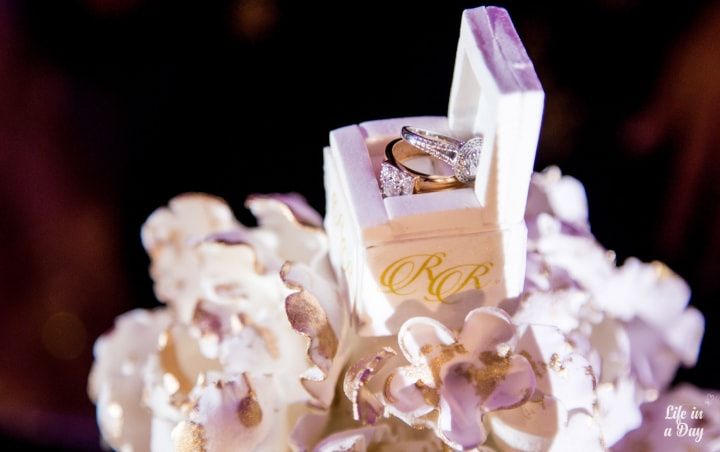The photograph presents a detailed close-up of an elegant, square-shaped white ring box with a subtle purple sheen, opened to reveal two exquisite diamond rings inside. The jewelry rests atop a cluster of soft, lilac and white, fluffy flowers, which may either be real or ceramic. Dominating the image, the floral base adds a delicate touch, suggesting it could be designed as a cake topper. The background is a solid, rich purple, ensuring no distractions from the central items. The box features two ornate, gold-scripted capital "R"s on its side. One of the rings is crafted from platinum or silver, showcasing a large circular diamond surrounded by smaller diamonds. The other ring appears to be a gold engagement ring with a prominent square diamond. Completing the image, the words "life in a day" are inscribed in white text at the bottom right corner, adding a contemplative nuance to the detailed and vibrant composition.